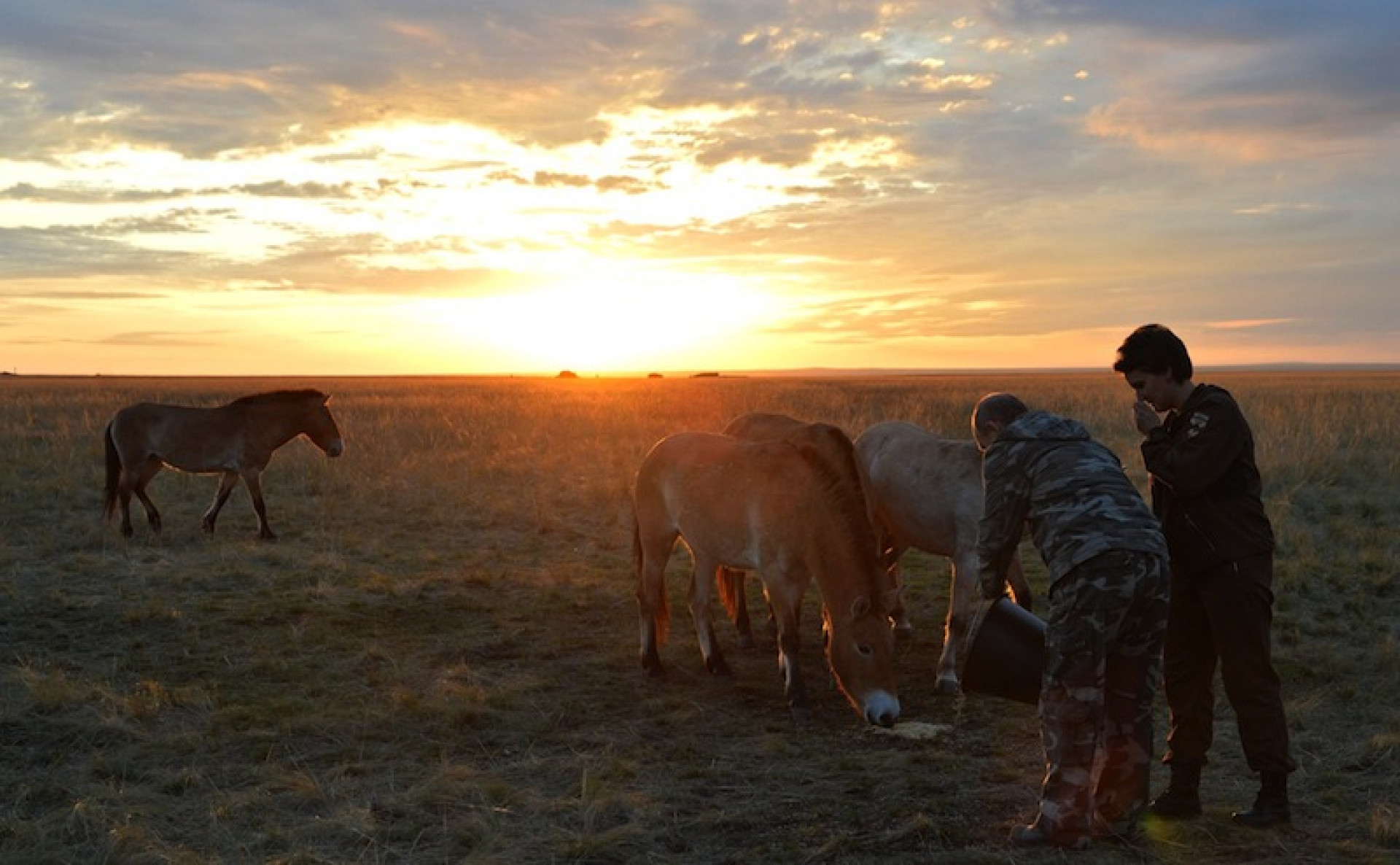In this detailed, photographic image taken in a horizontal landscape format during sunset, we see a serene outdoor field setting. The sky is a vibrant mix of shiny oranges near the horizon, transitioning to blue with white clouds higher up. In the lower right corner of the picture, there is a man dressed in a camouflage outfit, complete with a hood, as he leans over, pouring grain from a black plastic bucket onto the ground. Standing slightly behind him is a woman with short dark hair, clad in black military-style clothing and black boots. Her left hand is raised near her face.

In the foreground, two horses, one light brown and one white, are facing the camera and grazing on the ground where the man poured the grain. To the left, another darker brown horse walks into the frame, potentially moving towards the feed. The entire scene is bathed in the warm, glowing tones of the setting sun, adding a picturesque quality to this tranquil rural moment.